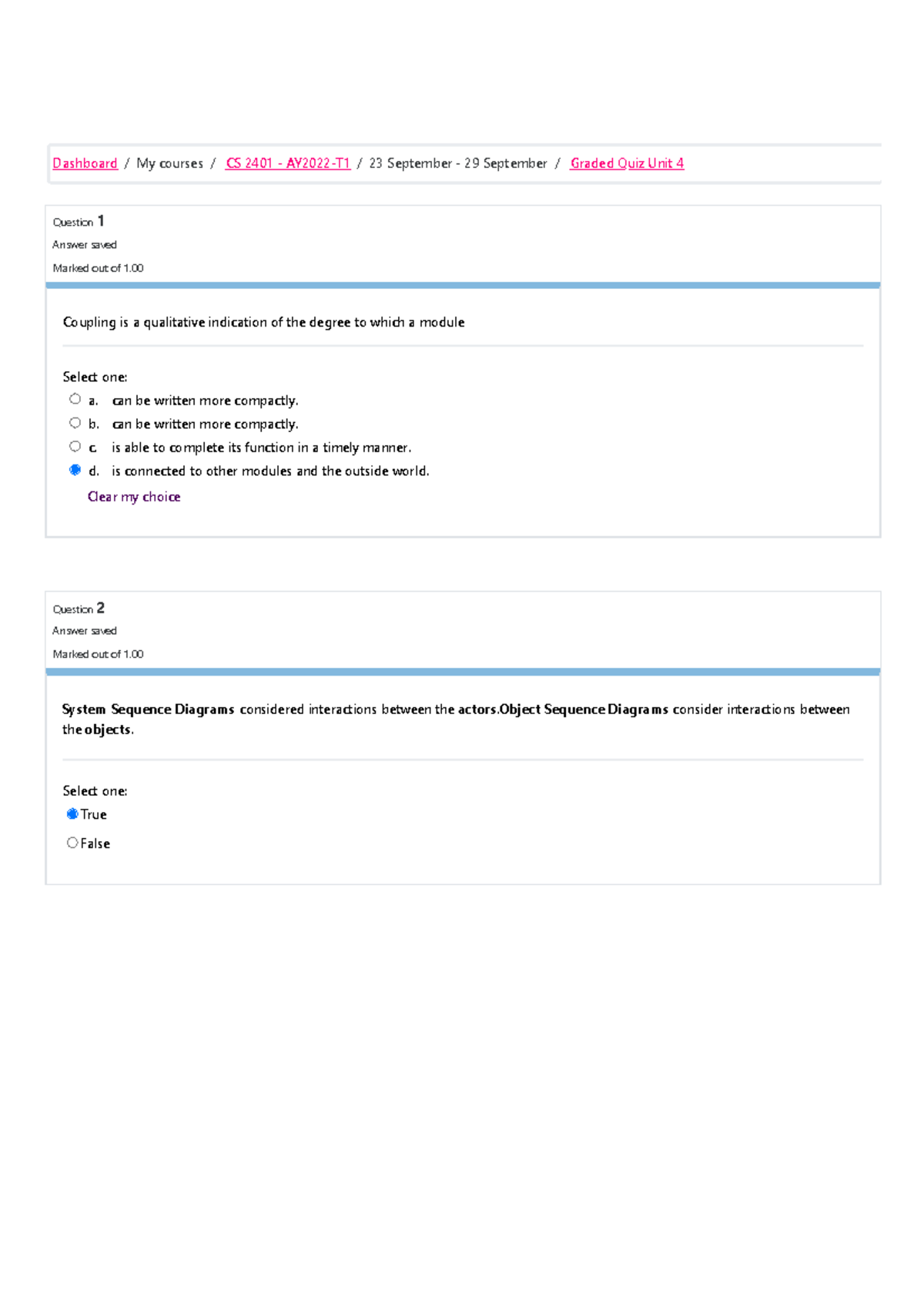The image depicts an online quiz interface for a course identified by the code "CX 2401" for Term 1, which spans from September 23rd to September 29th. The interface has a pink underline beneath "Dashboard" and "MyCourses," and the path indicates the specific quiz: "Graded Quiz Unit 4."

Immediately below the dashboard section, "Question 1" is written in bold. Below this, an answer box reads "Marks out of 1.00" with a horizontal blue divider separating the marks from the question text. The question displayed is: "Coupling is a qualitative indicator of the degree to which a model...," followed by a prompt to "Select one" from four multiple-choice options. The current selection is option D, which is highlighted in blue. There is a purple button labeled "Clear My Choice" that allows users to clear their selected answer.

Following this, "Question 2" is presented in a similar format: a bolded header "Question 2," an answer box with "Marks out of 1.00," another blue divider, and the question reads: "System sequence diagrams consider interaction between actors and objects." This question offers a true or false selection, with "True" currently selected.